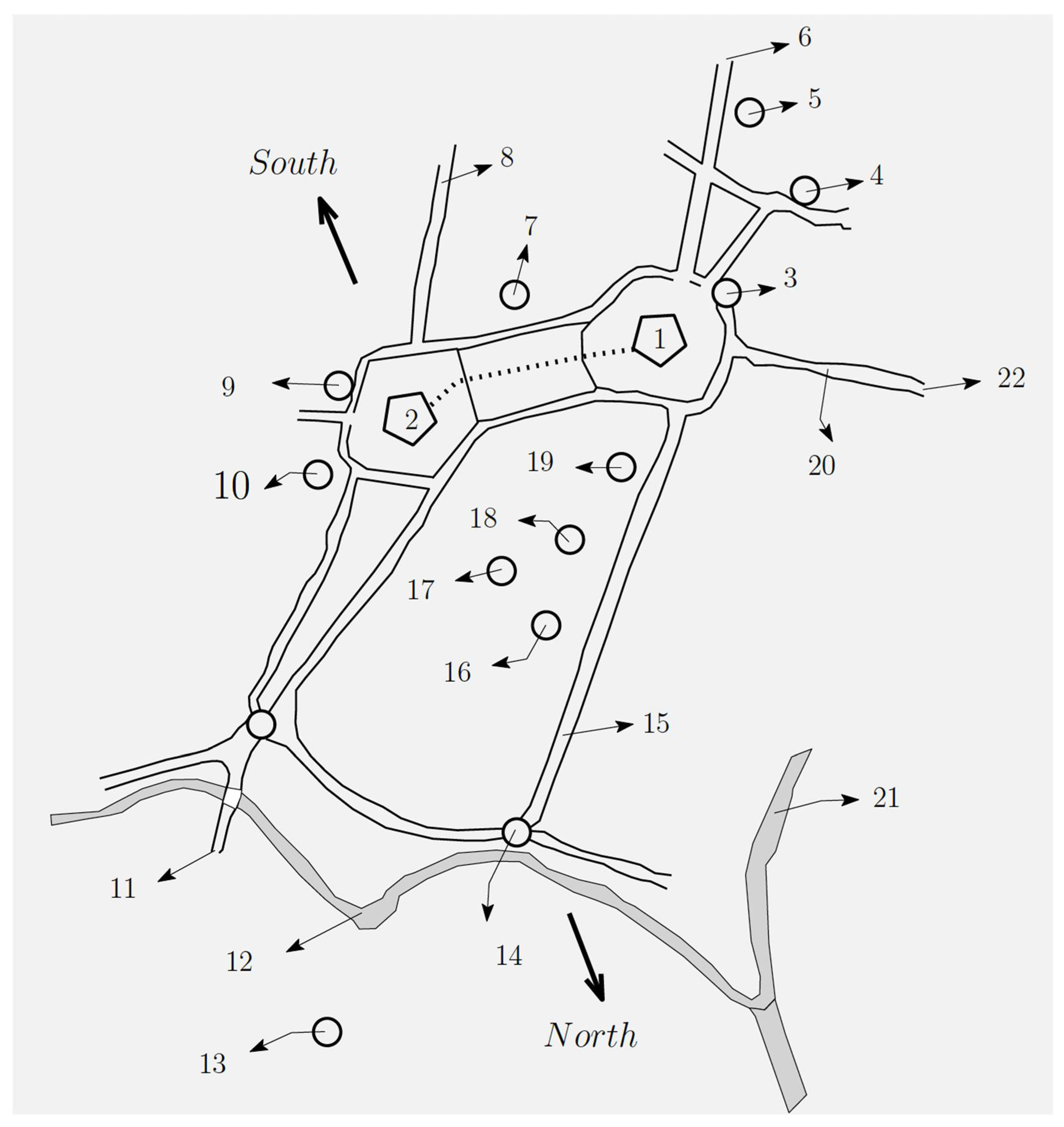This black and white photograph captures a detailed drawing of a map, potentially seen at a campground. It features a white background with various lines representing walkways and roadways. The map is annotated with the word "SOUTH" in black lettering at the top, accompanied by an arrow pointing toward the top left corner, and "NORTH" at the bottom with an arrow directed toward the bottom middle right. The central area of the map showcases two prominent numbers, 1 and 2, which are interconnected by dotted lines. Numerous arrows radiate from different circles labeled with numbers ranging from 1 to 22, indicating various sections of the map. These sections are represented by different shapes and sizes, branching out from the central area into smaller segments. Despite the clear layout, the map lacks a key or legend, leaving the specific purpose or destination of each number open to interpretation.